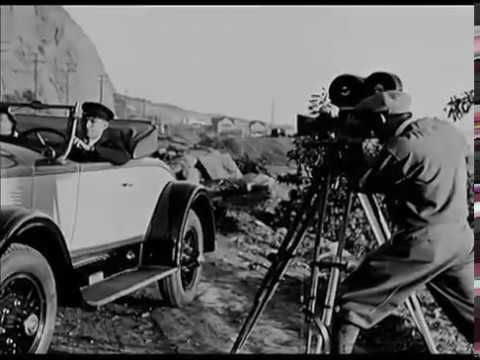The image is a black-and-white photograph capturing a scene reminiscent of an old-time movie set. In the foreground, a man dressed in a black suit and black hat drives a shiny, vintage convertible with the top down. The car features black spoked wheels and black fenders adding to its antique charm. Beside the car, on the left, stands another man in coveralls and boots, who appears to be operating a vintage film camera mounted on a tripod, complete with reels at the top. The action seemingly takes place next to a very old, dilapidated building along a rugged road. Though the distant background is unclear due to the lack of color and depth, hints of rocks and trees are faintly visible. The photo is horizontal and rectangular, with thin lines framing its corners, adding to the nostalgic feel of the composition. No explicit date is provided, but the attire, equipment, and overall scene strongly suggest a setting from a bygone era.